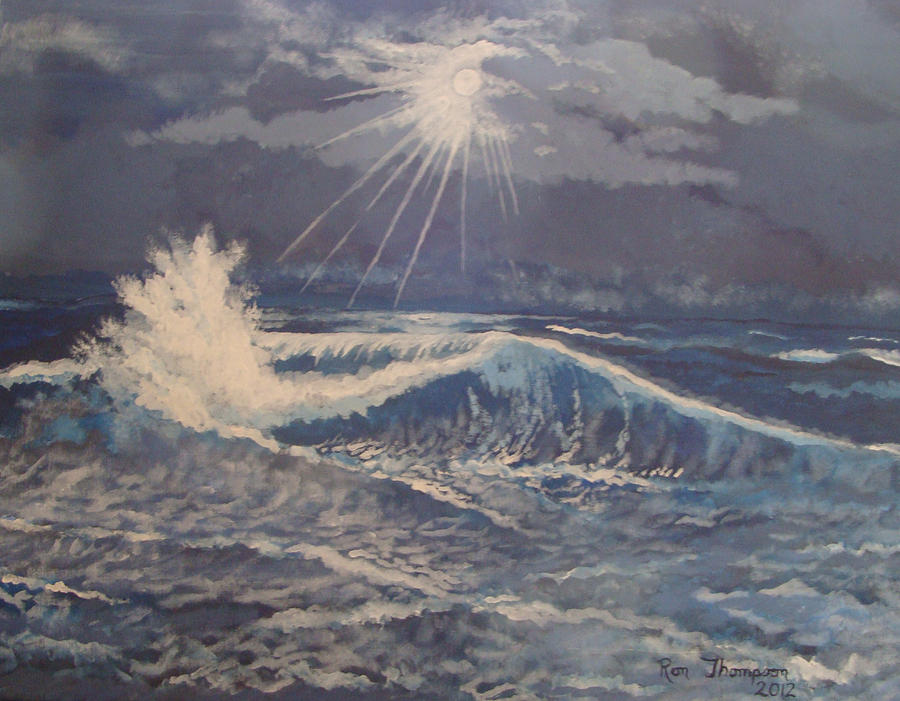This painting, created by Ron Thompson in 2012, vividly captures a dramatic seaside scene under an overcast sky. The canvas portrays a tumultuous ocean with waves crashing into each other, their frothy white tips highlighted with hints of gray. The sky above is a blend of dark and light gray clouds, with an enigmatic light source piercing through—a brilliant white that suggests either a strong moonlight or sunlight obscured by the heavy cloud cover. This light casts striking rays down onto the churning blue water, enhancing the sense of motion and natural power. The painting's composition, brushwork, and use of oil paints convey the raw beauty and restless energy of the sea, all subtly underscored by the artist's signature, "Ron Thompson 2012," neatly inscribed in the bottom right corner.